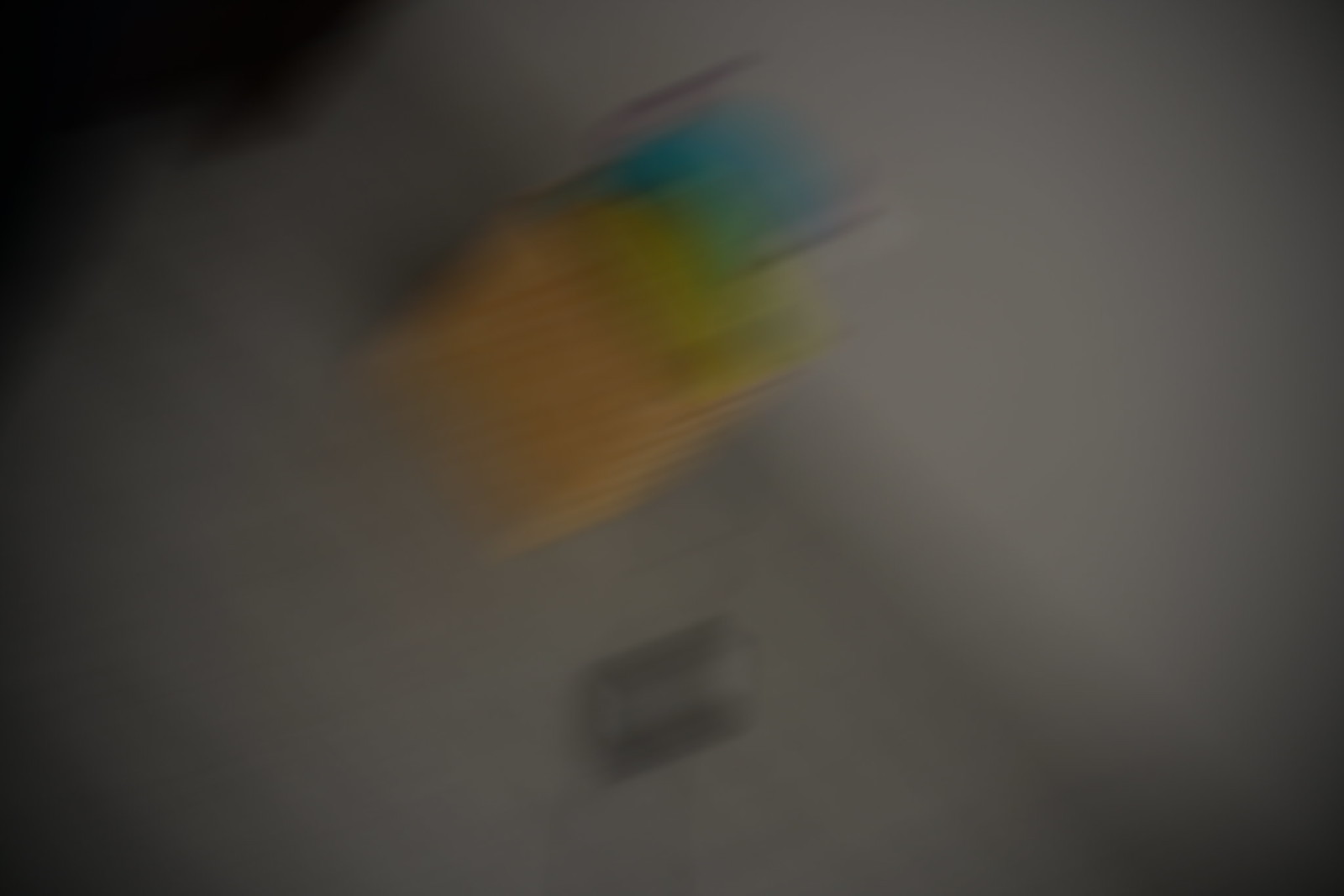This is a square-shaped, low-resolution image that is quite blurry and pixelated, making it difficult to discern specific details clearly. The central area of the image features indistinct shapes or objects. The color palette transitions from yellow at the bottom to green and then blue towards the top, creating a gradient effect. There is also a prominent black element below the central figure, though its exact nature remains unclear due to the poor image quality. The background of the image is a solid gray, devoid of any additional details or features.